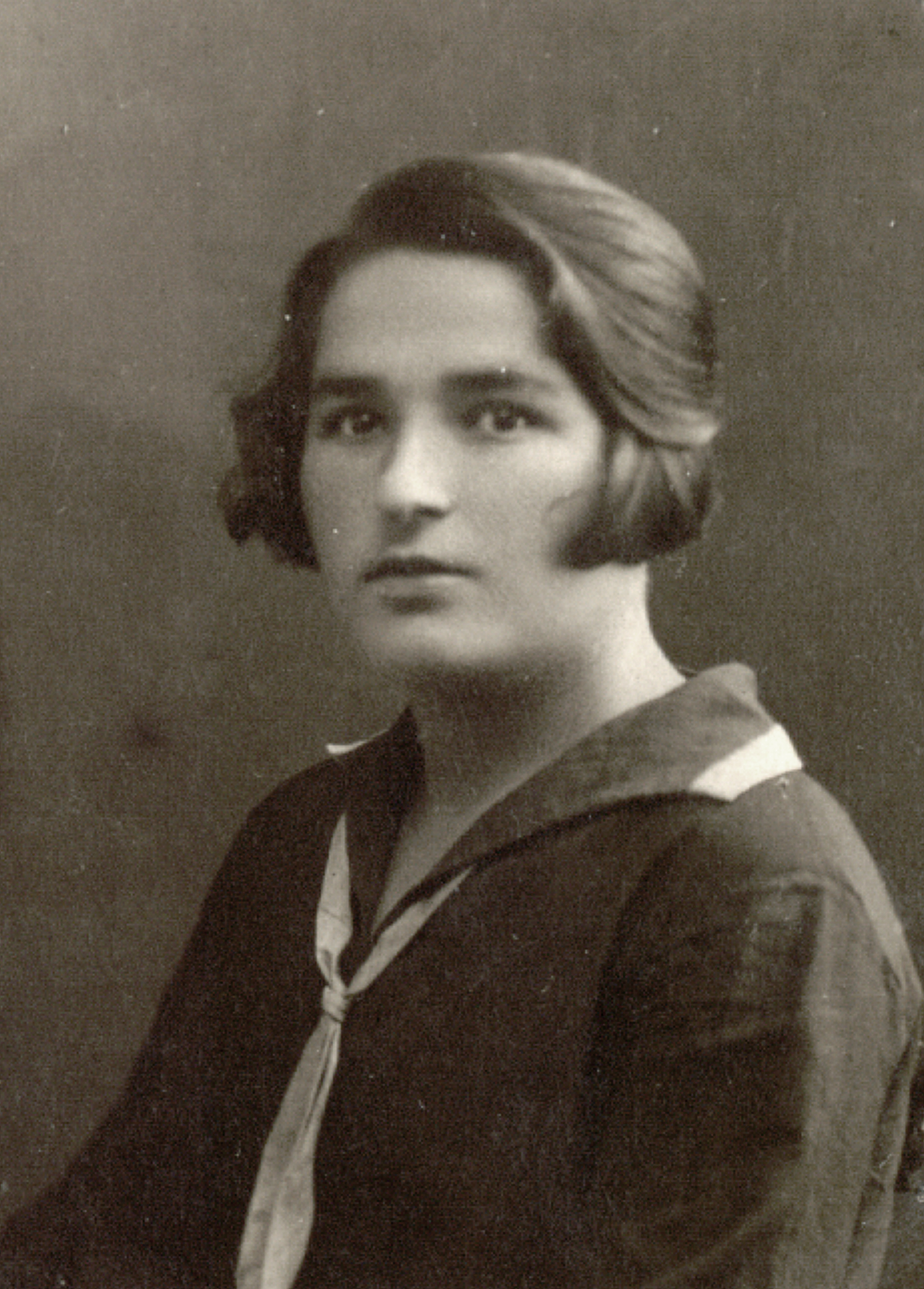This is a black-and-white portrait of a young woman with short, straight hair that slightly curls at the ends reaching down to her cheeks. Her bangs are pulled to the side, and her hair appears black in the grayscale image. She is wearing a long-sleeve black shirt with a loose-fitting v-neck collar, accentuated by a white scarf or handkerchief tied around her neck and hanging down her chest. The woman is facing forward, looking directly at the viewer with a neutral expression, her body angled slightly to the left. Her eyebrows are black, matching her hair. The background features a dark gray wall, which appears slightly lighter in the top left corner, giving an old-fashioned feel to the photograph. There are random nodes scattered across the image, indicative of its vintage quality and early 1900s style.